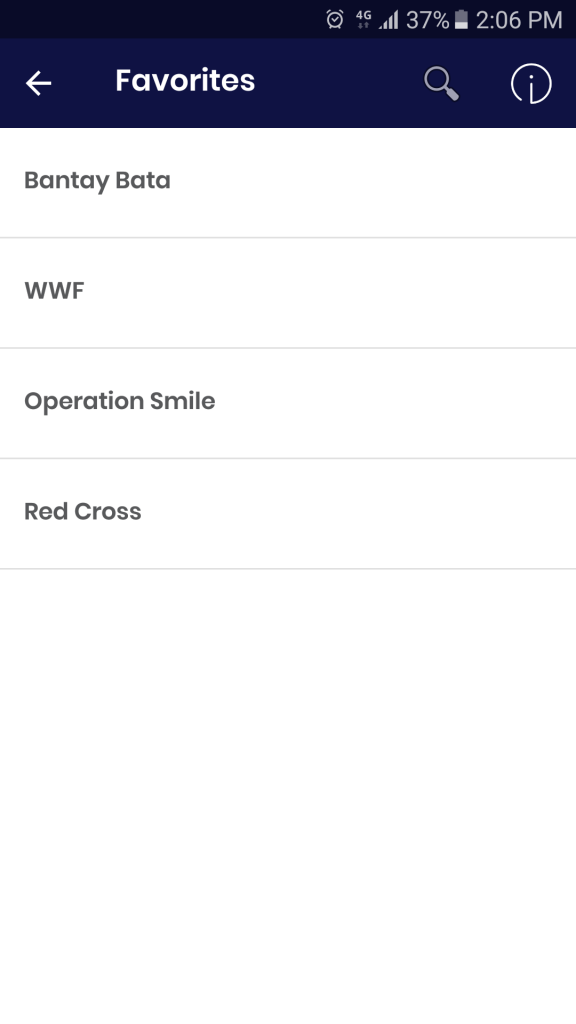In this image, we observe a cellphone screenshot displaying a curated list of favorite nonprofit or charitable organizations. At the very top, the phone's status menu is visible, indicating that this is indeed a screenshot. 

Beneath the status menu, a dark blue header with the label "Favorites" written in white prominently stands out. Below this "Favorites" header, there are four organizations listed sequentially in black font on a white background. These organizations are as follows:

1. Bantay Bata
2. WWF
3. Operation Smile
4. Red Cross

The list suggests that the individual who owns this phone has saved these organizations as their top non-profit or charitable preferences. 

The clean layout, with a clear white backdrop for the text, makes it easy to read and navigate. The use of a dark blue header helps in distinctly segregating the "Favorites" list from the rest of the phone’s interface.